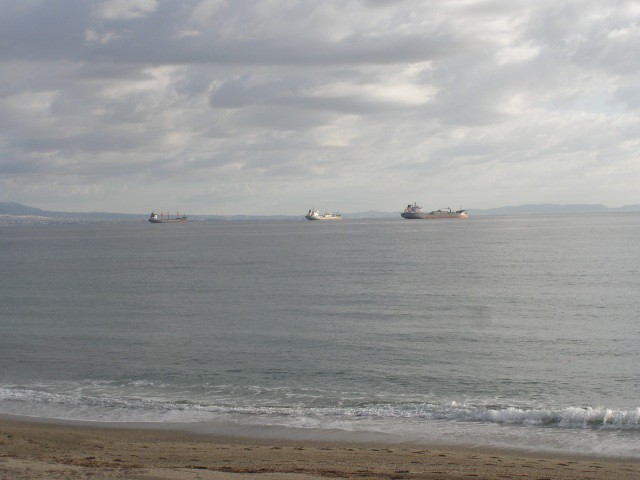The photograph, taken from the shore, presents a serene seascape with a well-groomed, sandy beach in the foreground. Small breakers ripple gently against the shoreline, indicative of the calm, peaceful water. Stretching to the horizon, the ocean dominates the middle part of the image, while the upper half showcases a light blue sky filled with scattered clouds, suggesting a partly cloudy day. 

Centered within this tranquil scene are three cargo ships, positioned in a three-quarter view with their bows pointing left. The ship in the middle is slightly smaller and white, while the larger ship to its right is gray. The leftmost ship appears gray with a white superstructure. The ships are too distant to discern specific details, but some vague features, such as poles or potential helicopter pads, are mentioned. 

Hints of a distant landmass, possibly islands or hills, can be seen faintly along the horizon, adding to the expansive depth of the scene. The entire composition suggests a calm day, devoid of heavy waves, and the soft lighting from the upper right creates a sense of gentle illumination across the image.